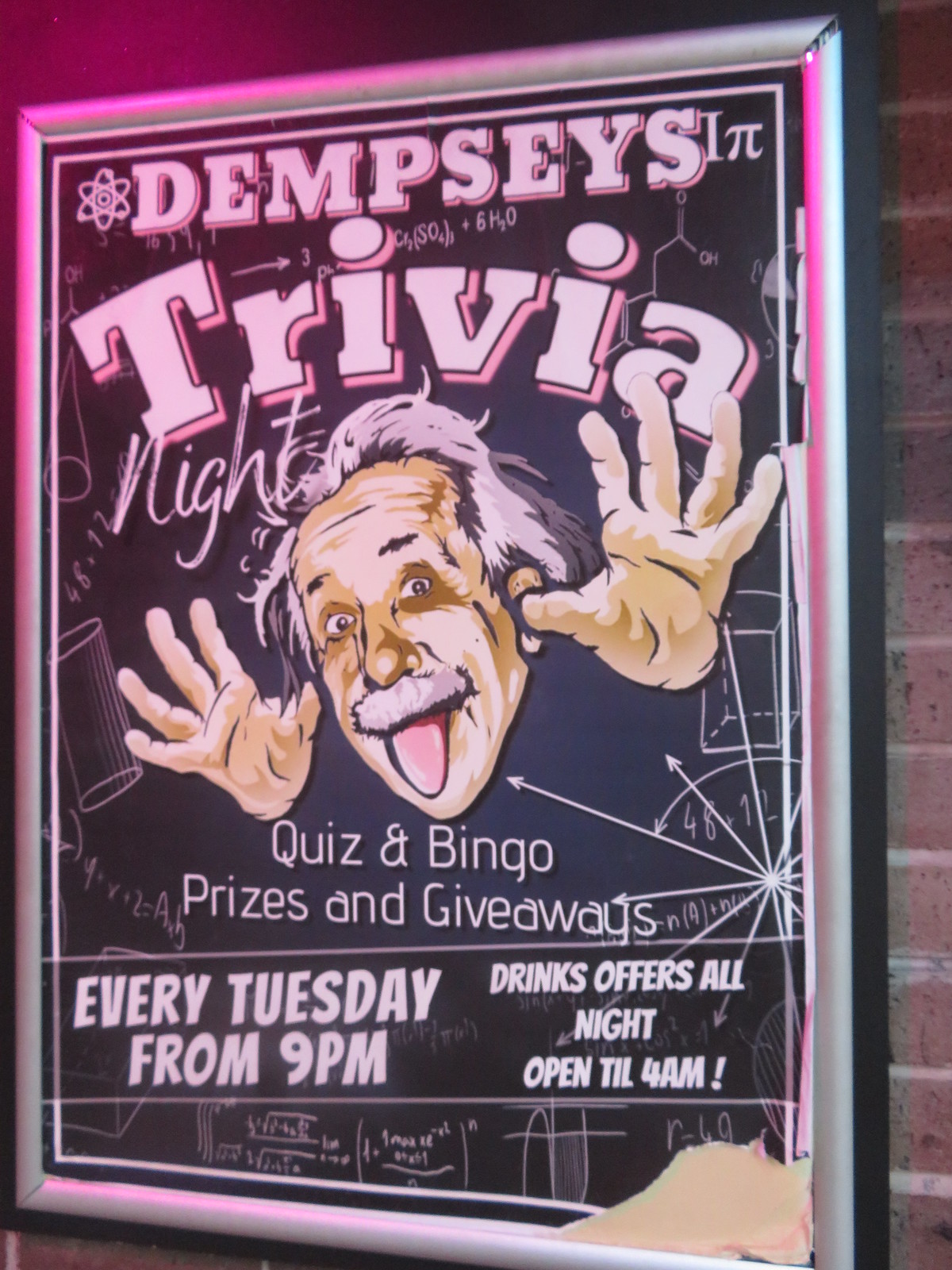This poster, promoting Dempsey's Trivia Night, is set against a brick wall and framed neatly in a black frame. Dominating the design is a lively, colorful illustration of Albert Einstein with his hands up and tongue out, exuding excitement and playfulness. Einstein is accompanied by a backdrop resembling a chalkboard filled with intricate math formulas, geometry patterns like cylinders, cubes, and rectangles, as well as graphs of various equations, all rendered in white chalk. This gives the poster a scholarly yet whimsical vibe.

Text details emerge prominently: "Dempsey's Trivia" is boldly announced at the top, followed by mentions of both quiz and bingo activities, with enticing notes about prizes and giveaways. Below, a small white box indicates that the trivia event takes place every Tuesday starting at 9 p.m., with drinks offered all night and the bar remaining open until 4 a.m. Adding a final touch, the poster is infused with a pink glow radiating particularly from the top left-hand corner, enhancing its eye-catching appeal.